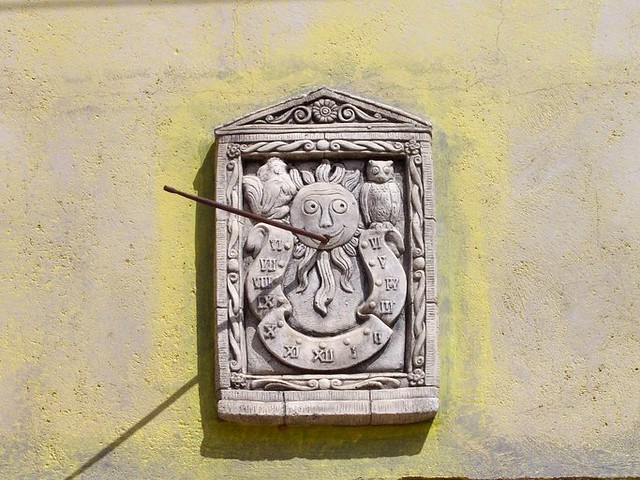This photograph features an intricately designed sundial mounted on a cream-colored stone wall. The sundial itself is either made of stone or crafted to resemble it, and it is framed by a brighter yellow border. Its shape consists of a rectangular base topped with a low, squat triangle, resembling a roof. The triangle is adorned with detailed engravings, including swirling patterns and a flower motif that extends down the sides and bottom of the sundial.

At the center of the sundial is a depressed circular section that features a sun with curving rays extending outward. The sun has a face with two eyes, a nose, and a smiling mouth. Emerging from the sun's mouth is a stick, whose shadow indicates the time on the sundial. Flanking the sun are two figures: a rooster to the left and an owl to the right, each meticulously crafted to add to the detailing.

Beneath the sun's face is a ribbon that winds up towards the left and right sides of the chin, adorned with Roman numerals indicating the hours the sundial measures. The background of the sundial is a textured, concrete gray, displaying natural imperfections like cracks and dents, which adds character to the overall composition. The shadow cast by the stick can be seen indicating the time, falling somewhere between the eight and nine o'clock marks.